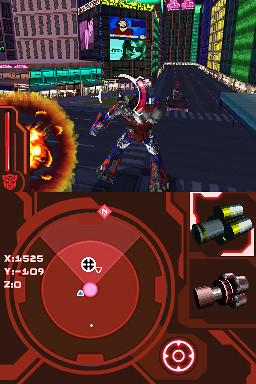This image, captured from a Transformers-themed video game, vividly features the iconic Optimus Prime prominently positioned at the top center, seemingly charging towards the camera. The lower portion of the frame displays a red map area denoting the player's current location. To the left middle of the image, a dynamic explosion is captured mid-blast. In the lower right corner, a selection of various gun styles is visible, indicating the player's weapon options. The backdrop is dominated by towering skyscrapers and an elaborate advertising structure reminiscent of Times Square. This structure showcases numerous large screens, including a newscast and an advertisement featuring a person wearing sunglasses. Below these digital displays, a series of storefronts line the street, adding depth and realism to the urban landscape.